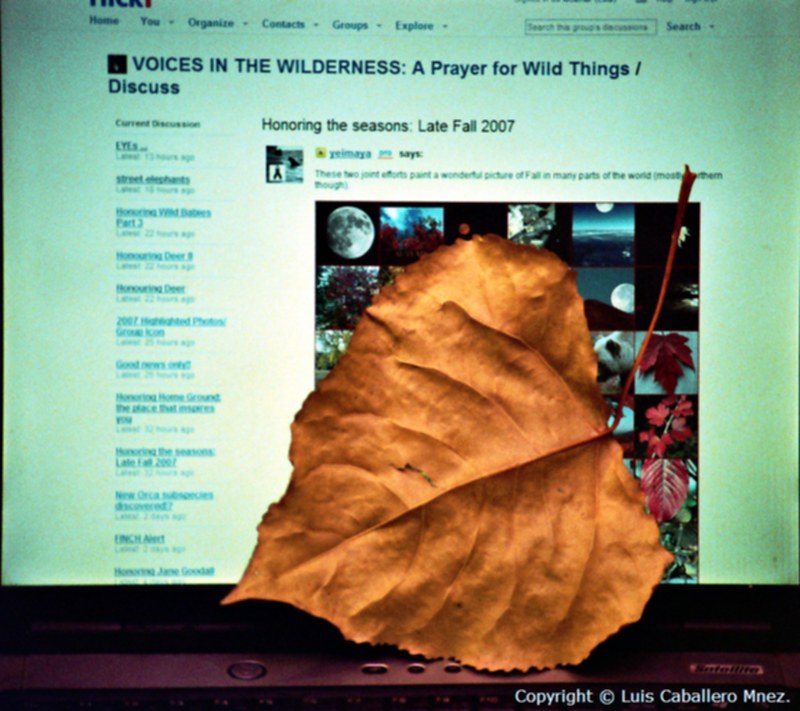The image depicts a computer screen, possibly a laptop or a monitor with a reflective gray border and buttons on the bottom. The screen displays what appears to be a webpage from the Flickr website. The background of the screen features a greenish-blue color with a prominent title at the top that reads "Voices in the Wilderness, A Prayer for Wild Things / Discuss." Below this, there's a subheading that says "Honoring the Seasons, Late Fall 2007." On the right side of the screen, there is a series of small fall-themed photos, and text columns are visible on the left side, though some details are obscured.

A noteworthy detail is a large, brown, heart-shaped leaf propped up in front of the screen. The leaf is crispy-looking, with visible veins and a slight crack that lets a small amount of light through, adding to its texture and detail. The leaf's stalk points upward, partially covering some of the images on the screen. Additionally, there is a copyright notice at the bottom of the screen that reads "Lewis Caballero MNEZ."